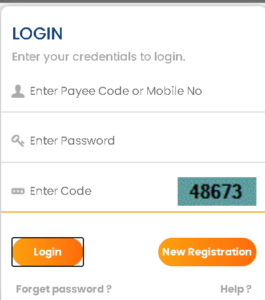Portrait-oriented image showcasing a login screen for an unknown program or website. The background is primarily white, framed by thick gray lines at the top and thin gray lines on the left side. 

At the top left corner, large blue text reads "Login." Below it, smaller gray text instructs users to "Enter your credentials to login." 

The first input area is marked by an icon of a person silhouette and the prompt "Enter payee code or mobile number," separated by a thin gray line. Following this is a key icon next to the prompt "Enter password," also divided by a gray line. Lastly, there's an icon too small to discern next to the prompt "Enter code," followed by a green box containing the numbers "4867300," separated by an orange line.

Below this, there are two orange ovals with white text. The first reads "Login" and has a black rectangular border around it. Adjacent to it, the second oval reads "New Registration." Under the "Login" button, there's a "Forgot Password?" link, and under "New Registration," a "Help" link is provided.

The login screen's purpose is not specified but appears to be for entering credentials on a website or program.